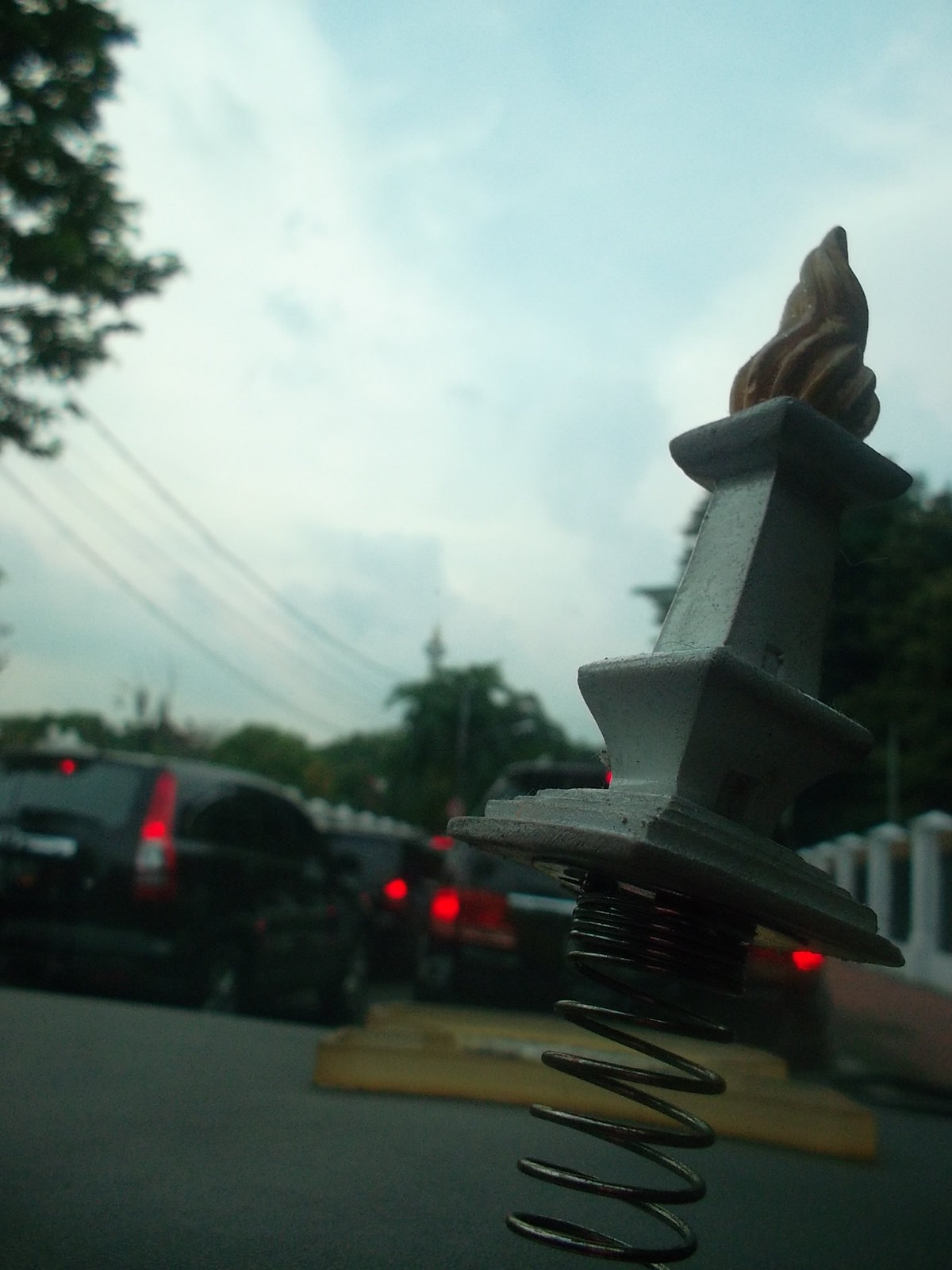The photo captures a bustling roadway, possibly a bridge, teeming with cars, hinting at a heavy traffic scenario. Despite the congestion, only three or four vehicles are clearly visible in the frame. Overhead, an array of phone lines crisscross the scene, while trees dot the landscape, framing the urbanized setting with a touch of nature.

At the center of the image stands a striking cement structure, bearing a decorative element that resembles a torch. This flame-like adornment, weathered with time, bears a brownish hue, evoking the appearance of a soft-serve ice cream swirl. The combination of natural and man-made elements creates a visually interesting contrast, capturing the essence of an urban environment mingled with natural surroundings.